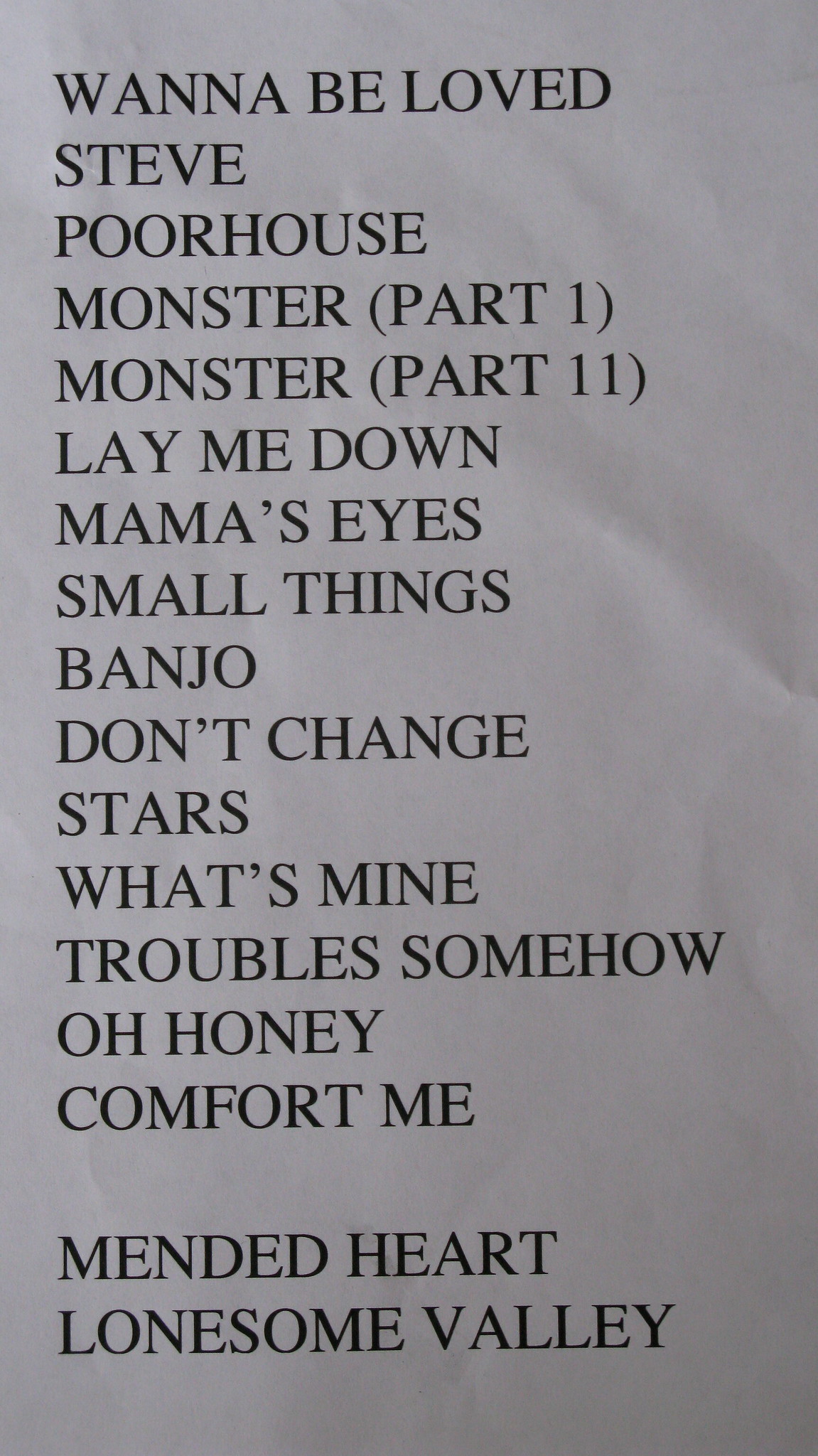The image is a tall, rectangular photograph of a slightly wrinkled, grayish piece of paper, displaying a setlist in black, all-capital letters. The paper appears white originally but is shaded gray due to shadows, and it has dents in the right middle and top right corner. The background is empty and unremarkable. The setlist from top to bottom reads:

WANNABE LOVED  
STEVE  
POOR HOUSE  
MONSTER (PART 1)  
MONSTER (PART 2)  
LAY ME DOWN  
MAMA'S EYES  
SMALL THINGS  
BANJO  
DON'T CHANGE  
STARS  
WHAT'S MINE  
TROUBLE SOMEHOW  
OH HONEY  
COMFORT ME  

After a space, it continues:

MENDED HEART  
LONESOME VALLEY